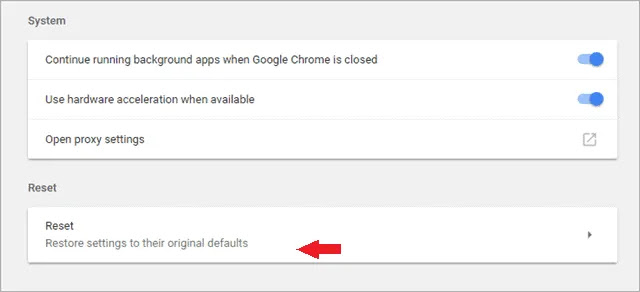This image showcases a section of Google Chrome settings, specifically focusing on system options and reset settings. The background is light gray, providing a subtle contrast to the white foreground of each section.

The first section titled "System" includes three options:
1. "Continue running background apps when Google Chrome is closed" - A blue toggle slider to the right indicates this option is enabled.
2. "Use hardware acceleration when available" - This also has a blue toggle slider to the right, showing it is enabled.
3. "Open proxy settings" - Accompanied by a gray, non-interactive icon of a box with an arrow pointing to the upper right, indicating this option is currently disabled or inactive.

Below the "System" section, there's another section titled "Reset." Within this section, there is a single option labeled "Reset," accompanied by a description that reads, "Restore settings to their original defaults." A prominent bright red arrow points towards this description, drawing attention to the reset functionality. On the far right of the "Reset" section, there is a triangle pointing to the right, suggesting this may be a clickable arrow, but it is not highlighted or activated.

The image effectively highlights important settings within Google Chrome, particularly drawing focus to the reset option, which is emphasized by the bright red arrow.